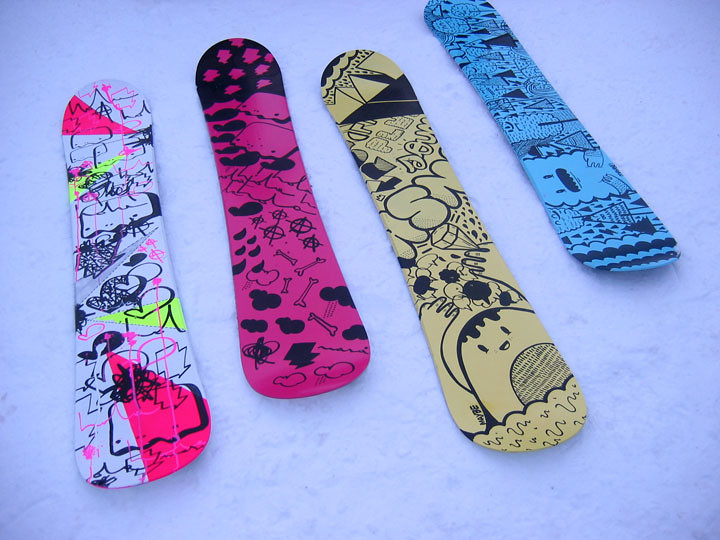A vibrant and detailed image of four snowboards, lying flat on sparkling white snow, facing roughly the 11 o'clock position. The background snow appears slightly melted with a higher blue hue, featuring subtle cracks but remaining largely trackless. The board on the left showcases a white base with hot pink and neon yellow areas, along with black heart shapes and random black lines. Next to it, a snowboard with a hot pink backdrop is adorned with black storm clouds, dog bones, two dogs, and rain. The third one stands out with a banana yellow color, featuring a cartoonish donut character with raised hands, a diamond in one hand, a pair of scissors at the top symbolizing a storm, and some bubble letters. The board on the far right is baby blue, detailed with various black and textured triangles, a fried corn dog, smiley-faced meatballs, and a screaming cloud towards the bottom.